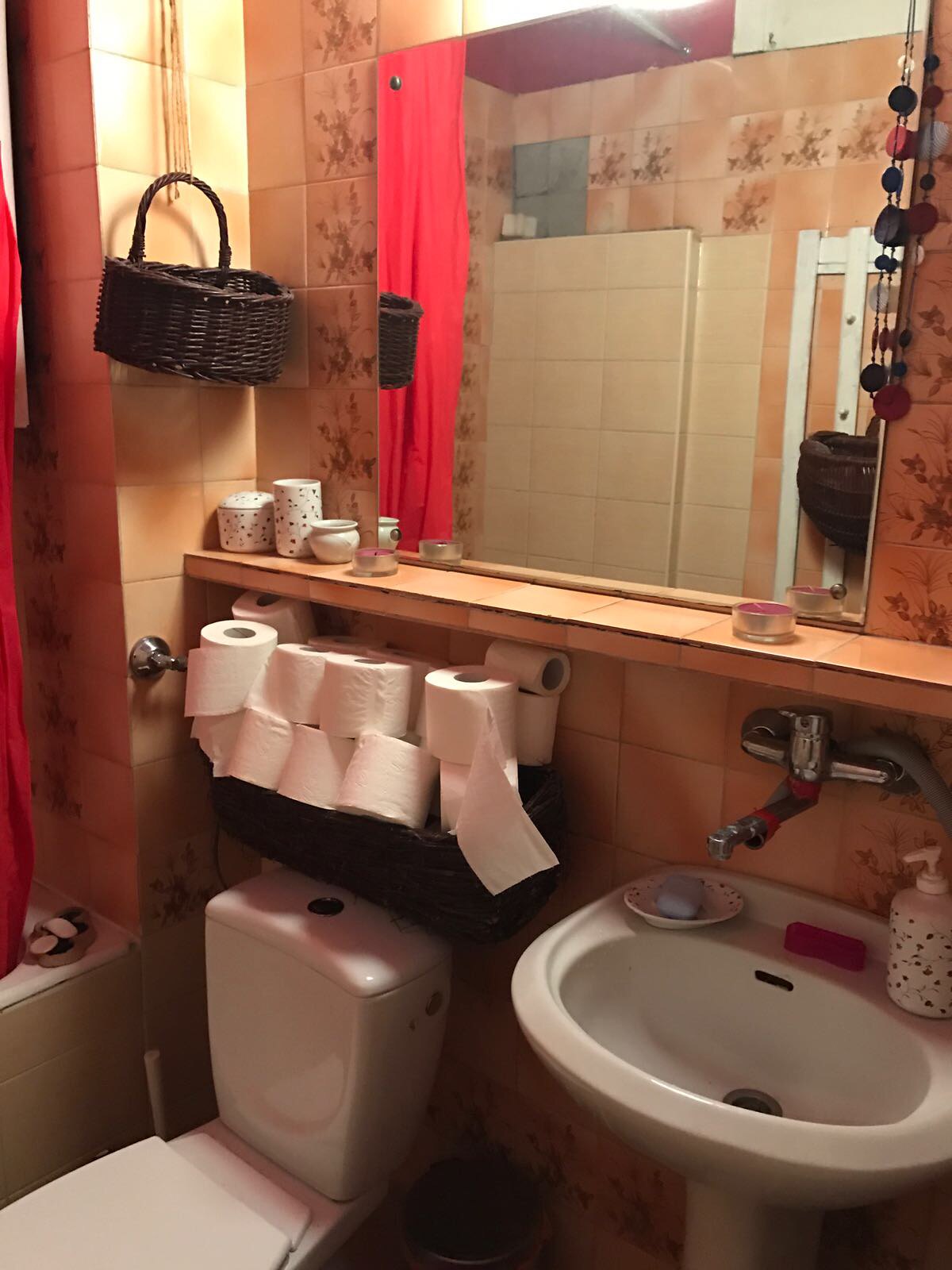The color photograph captures a bathroom bathed in a magenta, pinkish tint from artificial lighting. Central to the scene is the lower left-hand corner featuring a porcelain toilet, crowned with a rectangular dark basket haphazardly filled with around twenty rolls of toilet paper, some appearing used and of varying sizes. Above the toilet, on the wall, hangs a square mirror, adorned with a necklace on its right, reflecting the tiled wall from the opposite side of the room. A notable red shower curtain can be seen hinting at a tub in the background. To the bottom right, a white porcelain sink is prominently displayed, equipped with a silver wall-mounted faucet. On the sink, there is a round white soap dish adorned with different colored specks, holding two soap bars—one blue and one red—and a liquid soap holder. The tiled wall extends consistently across the image, juxtaposing the neatness of the sink area with the organized chaos of the toilet paper basket.